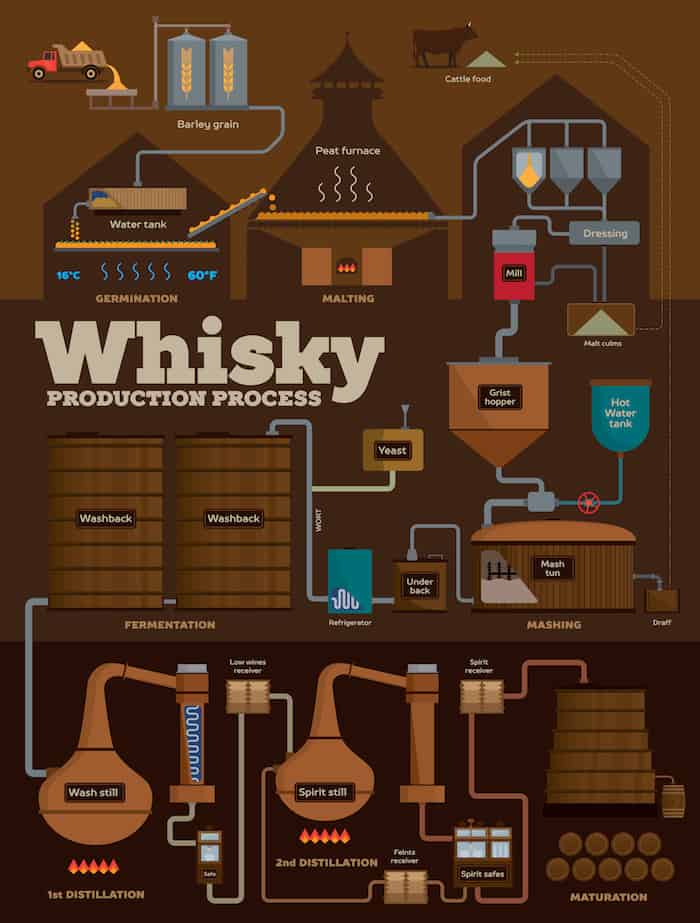The image titled "Whiskey Production Process" is a vertically aligned rectangular diagram with a predominantly brown background featuring various shades of brown, as well as accents of white, aqua, red, yellow, and light green. Starting from the upper left corner, the process initiates with a dump truck emptying barley grain onto a container from which pipes transport the grain to two labeled silos. Another pipe directs the barley to a water tank, signifying the germination process, which occurs at temperatures between 16 degrees Celsius and 56 degrees Fahrenheit. The conveyor valve moves the grain to a peat furnace for malting. An icon of a cow next to the furnace indicates that the by-product, cattle food, is generated here.

Continuing downwards, the diagram includes stations labeled malting, MRI, and dressing, along with a grist hopper and a hot water tank. Icons guide the viewer through various steps, such as a mash tun and an underback, which are critical components in the mashing process. The incorporation of yeast follows, depicted by a small box, and the mixture flows into a washback tank. Subsequently, the wash enter wash stills and spirit stills, marked by first and second distillation stages, which are signified by flame icons. 

Finally, the spirit travels into barrels for the maturation process, indicating the whiskey is aging over time. The entire diagram, accented with colors, outlines the detailed journey from barley grain to matured whiskey in a visually engaging manner.